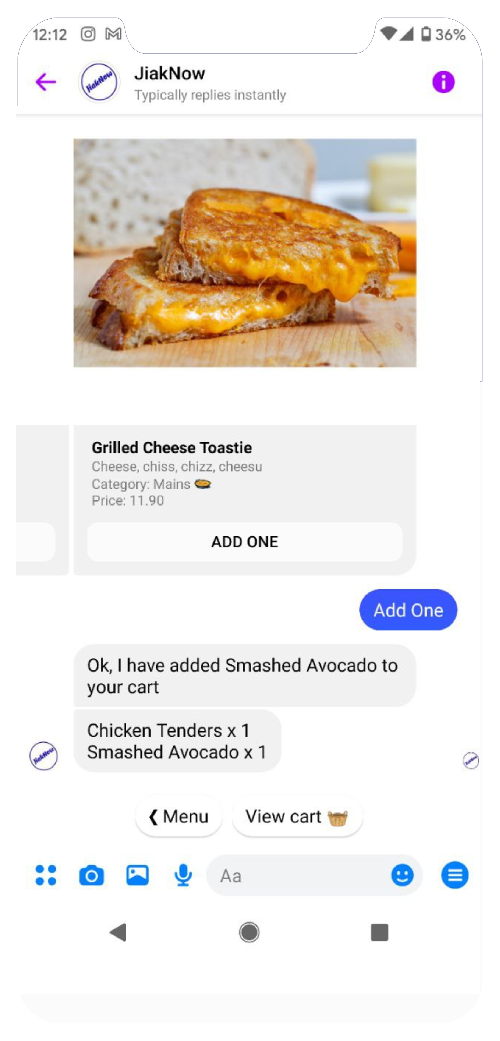**Descriptive Caption for Screenshot:**

This image is a detailed screenshot taken from a cell phone at 12:12 PM, as indicated by the time displayed at the top left corner. On the top right, the battery level shows 36%. Below the phone's status bar, the webpage's top banner features the website name "JakeNow" (spelled J-I-A-K-N-O-W) as a single word, followed by the tagline “typically replies instantly.”

Prominently featured in the middle of the screenshot is a mouthwatering picture of a grilled cheese sandwich, neatly cut in half and artfully stacked. The sandwich rests on a wooden cutting board, with a loaf of bread halved and placed behind it, serving as a picturesque backdrop.

Beneath the image, text describes the dish as a "grilled cheese toasty" with a playful repetition of the word "cheese" in various quirky spellings, including "cheese, cheese, cheese, cheese, cheese, cheese, cheese, cheese and cheesu (C-H-E-E-S-U)." This dish is categorized under the mains and priced at $11.90. Just below, two buttons allow users to add the item, each labeled "Add One."

Further down, a notification confirms, “Okay, I have added smashed avocado to your cart.” The cart contents show "Chicken tenders, times one” and "Smashed avocado, times one." Two action buttons at the bottom facilitate navigation: "Menu" and "View Cart."

Finally, at the very bottom of the webpage, there are navigation icons enabling users to take a picture, post a picture, upload a picture, or send a message.

Note: This detailed description adds clarity and context to the elements visible in the screenshot, providing a comprehensive understanding of the content.